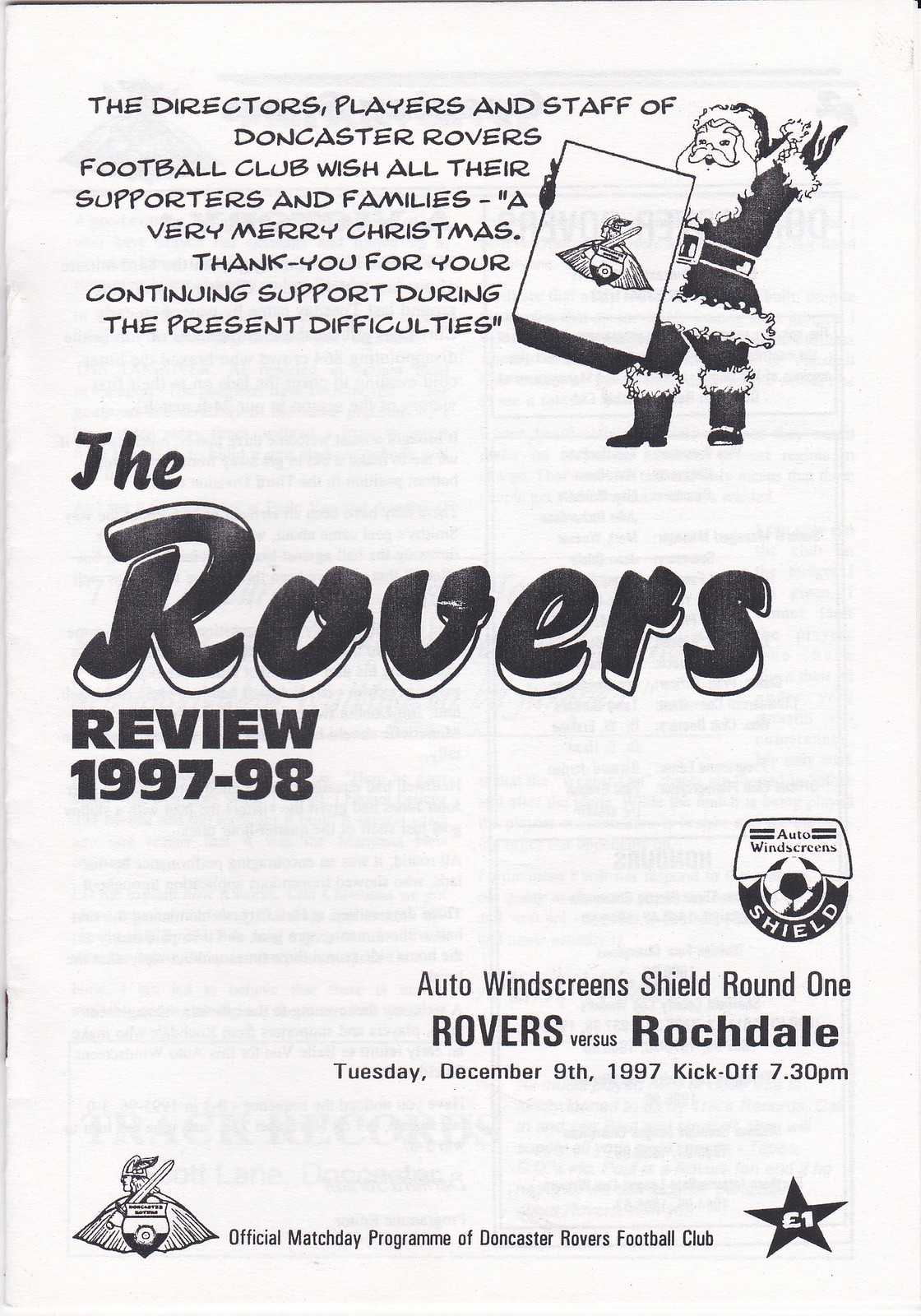The image is the front cover of an official match day program for the Doncaster Rovers Football Club, titled "The Rovers Review" for the 1997-1998 season. The layout features a black and white design with a prominent cartoon of Santa Claus holding a sign with the club's logo in the top right corner. The top of the cover carries a festive message from the directors, players, and staff of the Doncaster Rovers Football Club, wishing their supporters and families a Merry Christmas and expressing gratitude for their ongoing support during challenging times. Below this, the program details the first round of the Auto Windscreen Shields, featuring a match between Rovers and Rochdale, scheduled for Tuesday, December 9th, 1997, with a kickoff time of 7.30 pm. The bottom of the cover includes additional club logos and a star indicating the price of one pound.